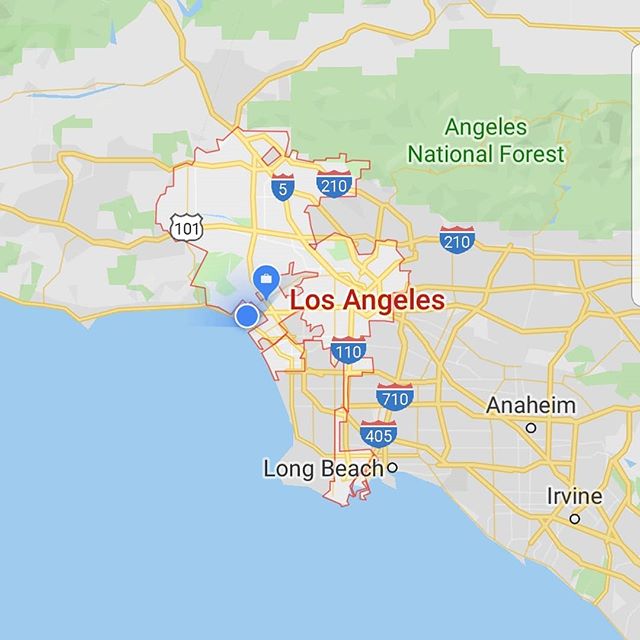This detailed map of Los Angeles prominently features the city's intricate network of highways and streets. Central to the image, Los Angeles is highlighted in red, indicating it as the main focal point. Key highways such as the 110, 710, and 405 are marked with distinctive upside-down blue triangles containing their respective numbers. Surrounding the Los Angeles area to the south, locations like Long Beach, Anaheim, and Irvine are visible, while the Angeles National Forest dominates approximately 30% of the map's top section.

The highlighted Los Angeles area is outlined in red, stretching from the 210 highway above the city, intersecting with major routes like the 5, 210, and 101, extending down towards Long Beach. Green patches sporadically mark nature-based sites, and general land areas are shaded in gray. Above each highway marker, three red lines mimic the standard highway symbol for easy identification. 

Additionally, a blue raindrop-shaped marker indicates a specific location of interest, possibly the map's owner's workplace, while another marker subtly suggests the viewer's current location, positioned just to the left of the Los Angeles label on the map.